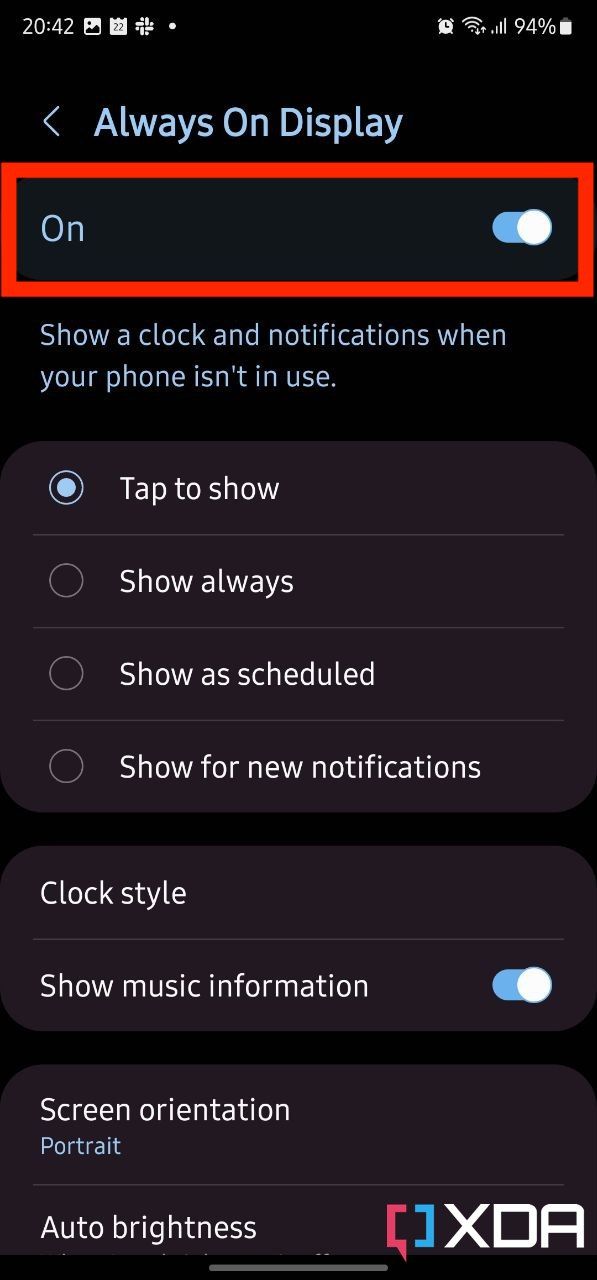Screenshot of a mobile device with a black background. At the top left corner, the time reads 20:42, accompanied by various notifications. On the top right, indicators show that an alarm is set, Wi-Fi is active, cell signal is maxed out, and the battery is at 94%. Below this, the main content displays the "Always On Display" settings menu. The slider switch for the "Always On Display" feature is set to "On," highlighted by a red box. The text below the slider reads, "Show a clock and notifications when your phone isn't in use," with options for customizing the display settings including "Show always," "Show as scheduled," and "Show for new notifications." Further down, "Clock style" and "Show music information" options are visible, with the latter turned on. Additional settings include "Screen orientation," set to portrait, and "Auto brightness." At the bottom of the screenshot, there is a watermark with a half blue, half red circle, and the text "XDA" beside it.